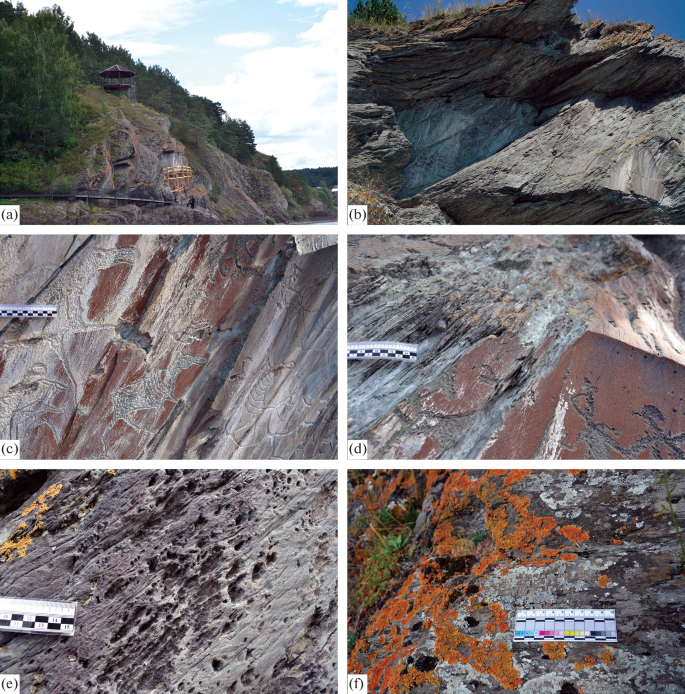The image is a collage of six outdoor daytime color photographs, arranged in two columns and labeled A through F from top to bottom, left to right. Each photograph showcases different aspects of a mountainside or hillside, emphasizing the rugged rock formations, intricate carvings, and varying vegetation.

Photo A reveals a mountainside covered in lush greenery, with an observation post and a pathway leading to a sheer cliff face. A building or water tower is visible nearby, adding a touch of human presence to the natural setting.

Photo B offers a close-up of the jagged cliff face, featuring an overhang and a mix of stone colors. The rugged texture of the rocks is immediately evident.

Photo C displays an intricately carved section of a smooth, weathered stone surface. The carvings include figures of animals, fish, and people, etched into gray and red stone. A small black and white ruler in the upper left corner provides scale.

Photo D focuses even closer on the stone carvings, highlighting the transition from red to brown to gray tones in the rock. The surface appears porous with smoothly rounded edges.

Photo E captures a heavily pot-marked, two-toned gray stone area. The surface texture resembles melted ice, further emphasized with the inclusion of a ruler for scale.

Photo F showcases a section of gray and brown rock, partly covered with green vegetation. An orange moss or lichen growth spans a large portion of the rock, adding a vibrant natural detail to the rugged scene.